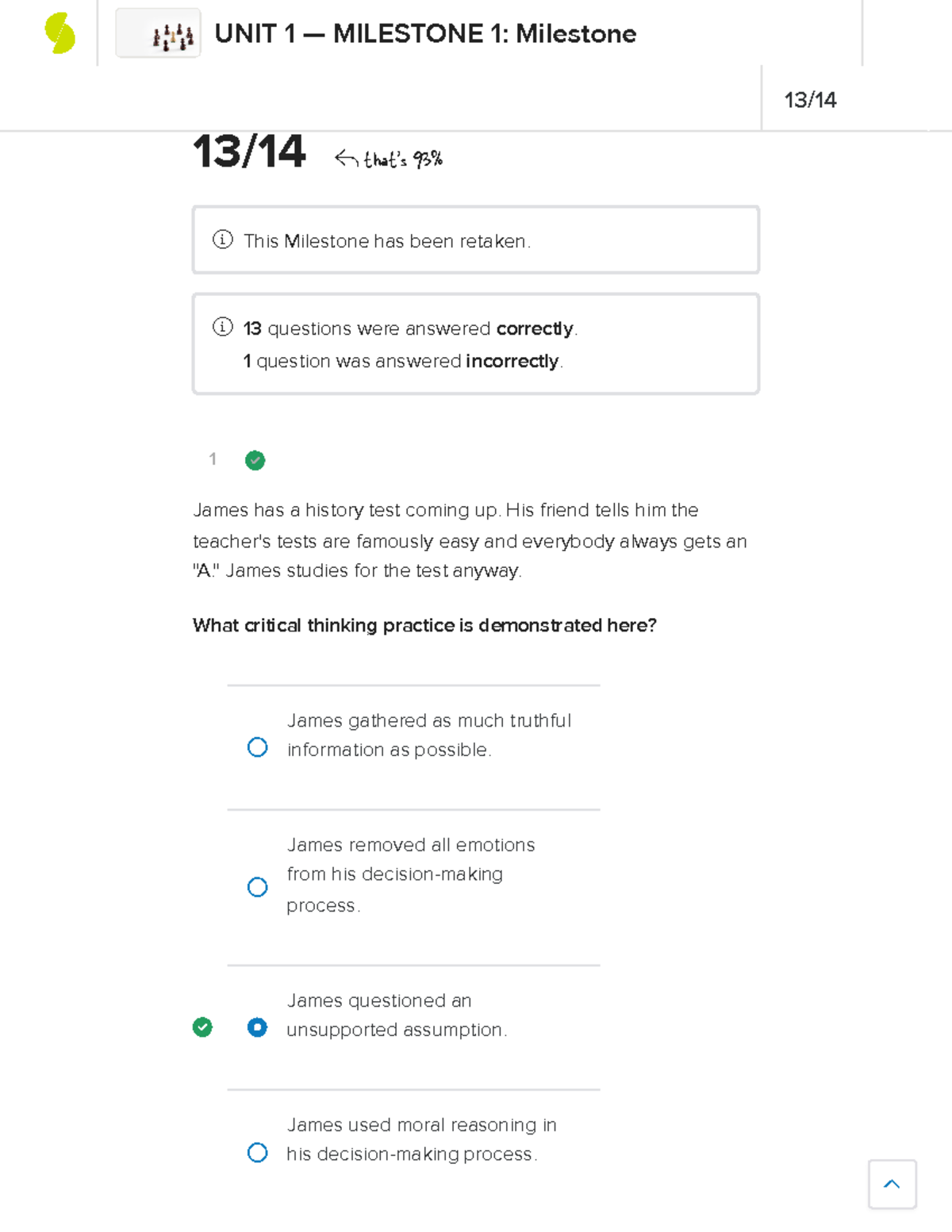**Detailed Caption:**
The image appears to be a screenshot from a mobile device, displaying academic progress within an online learning platform. The background is predominantly white. In the upper left corner, there are two lime green half circles with their flat ends facing each other but slightly misaligned. To the right of this icon, the text reads "Unit One Milestone One Milestone." On the far right of this section, there is a score displayed as "13 out of 14."

Below this section, still on a white background, the text again states "13 out of 14" with an arrow pointing to it and an accompanying note that translates this score to "93%." Directly beneath, there are two rectangular boxes. The first box states, "This milestone has been retaken," and the second box informs, "13 questions were answered correctly. One question was answered incorrectly."

Proceeding further down the screenshot, a test question from the milestone is visible. It reads: "James has a history test coming up. His friend tells him the teacher's tests are famously easy and everybody always gets an A. James studies for the test anyway. What critical thinking practice is demonstrated here?" Below the question, four multiple-choice answers are provided:
1. James gathered as much truthful information as possible.
2. James removed all emotions from his decision-making process.
3. James questioned an unsupported assumption.
4. James used moral reasoning in his decision-making process.

The individual selected the third option, "James questioned an unsupported assumption," which is marked with a green circle containing a checkmark, indicating the correct answer.